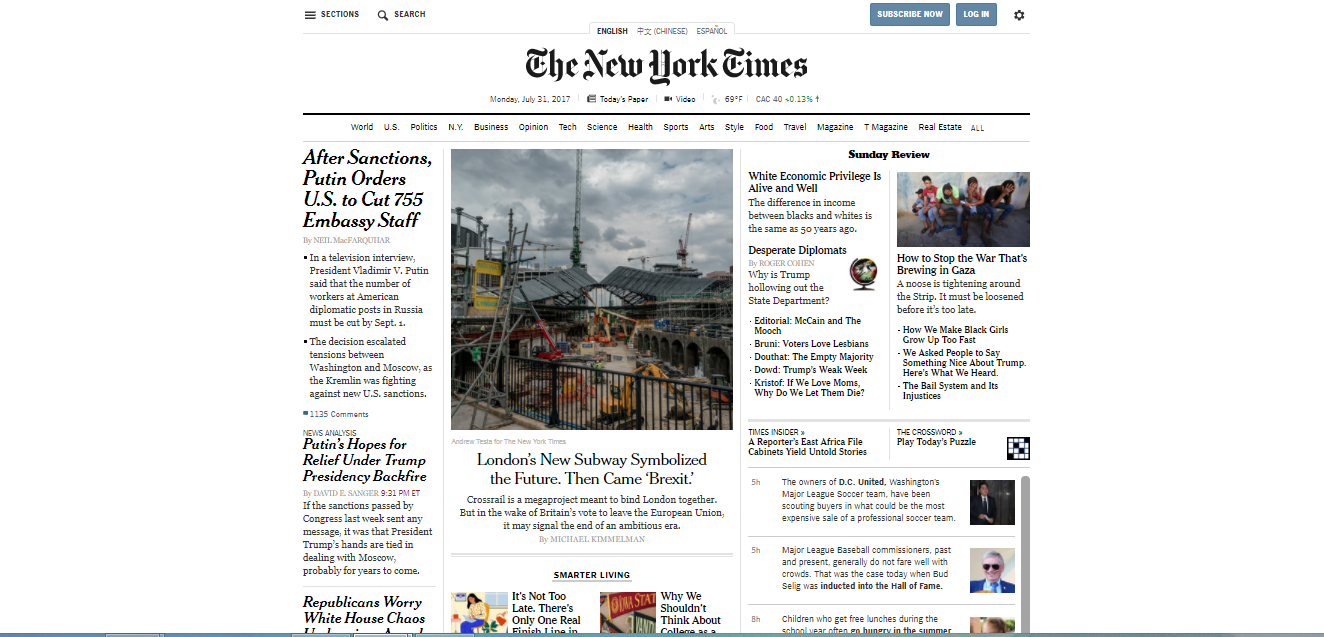This image showcases the front page of the New York Times web edition dated Monday, July 21st, 2017. The prominent header features a white background with the iconic New York Times logo rendered in the distinguished Times Roman font. Centered just below the header is a photograph depicting a scene under gray skies. In the foreground, a black metal fence is visible, alongside nearby buildings. The headline accompanying the photo reads, "London's new subway symbolized the future. Then came Brexit." To the left, another headline states, "After sanctions, Putin orders U.S. to cut 755 embassy staff." On the right side, additional headlines are visible, including, "White economic privilege is alive and well" and "Desperate diplomats."